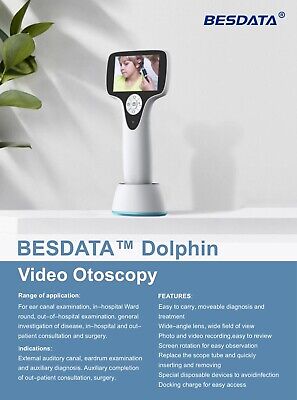The full-page magazine advertisement for the Best Data Dolphin Video Otoscopy prominently features the handheld otoscopy device at the top. The device has a sleek white base and a black screen, and it rests on a round white charger with a blue base. This setup leans against a white wall on a white table, with the partial view of a decorative plant's leaves to the right. The top right corner of the ad displays the Best Data logo. At the bottom of the image, a white rectangular strip boldly states "Best Data Dolphin," followed by a blue rectangular box with the heading "Video Otoscopy" and the product's benefits listed below. The image on the device screen shows someone examining a child's ear, emphasizing its use for ear health assessments.